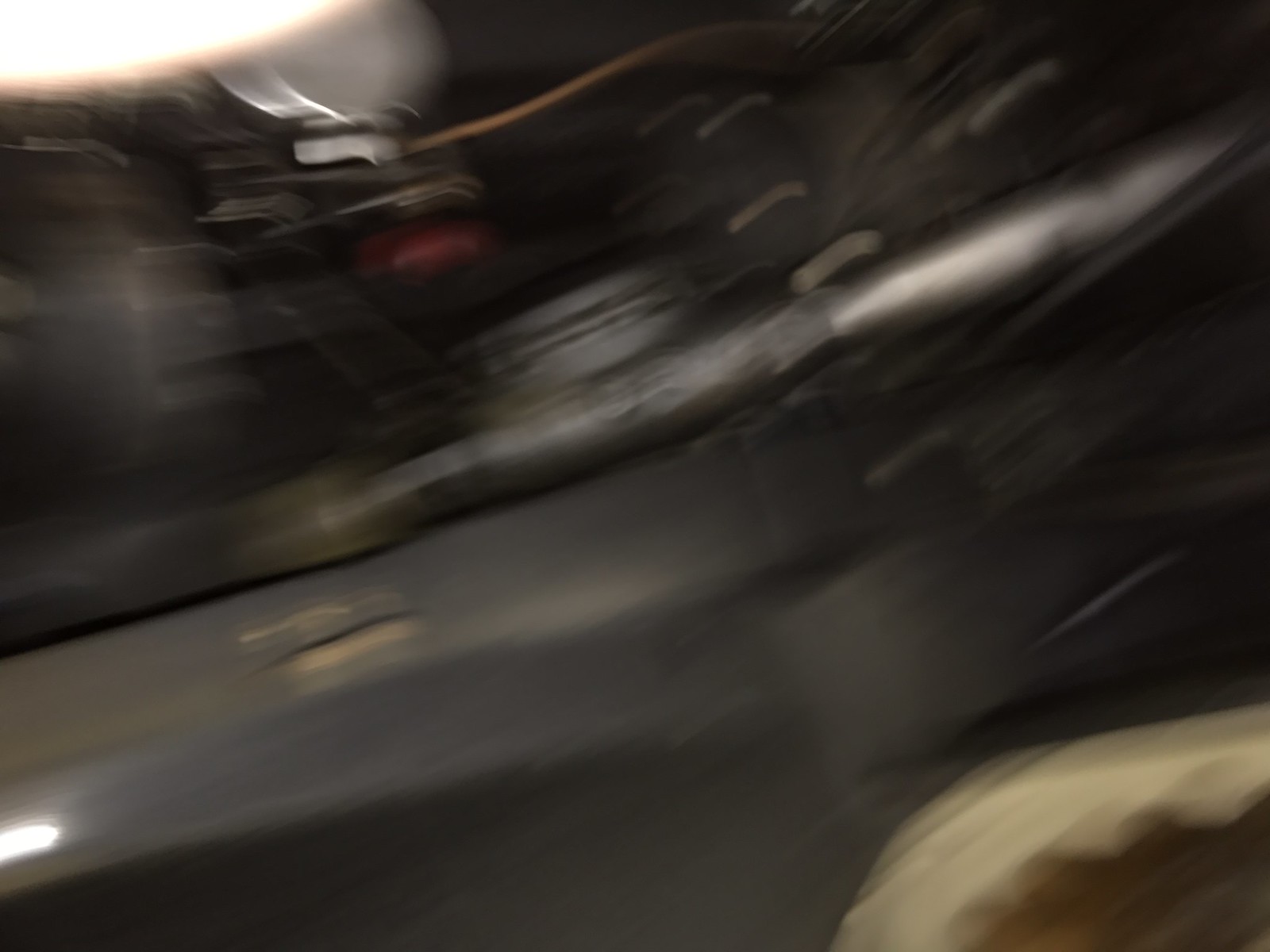This very blurry image shows a predominantly gray background with varying shades running throughout. In the bottom right corner, there's a patch of olive yellow color, while the top right corner is noticeably darker, approaching black. The middle of the image is more ambiguous but features a horizontal silver pipe running from left to right, turning grayish halfway across. At the upper left corner, there's a bright spot that stands out, along with a round silver piece beneath it. A brown piece of wiring can be seen stretching across the right side of the image. The overall blurriness suggests it may have been taken while in motion, thus making finer details challenging to discern.